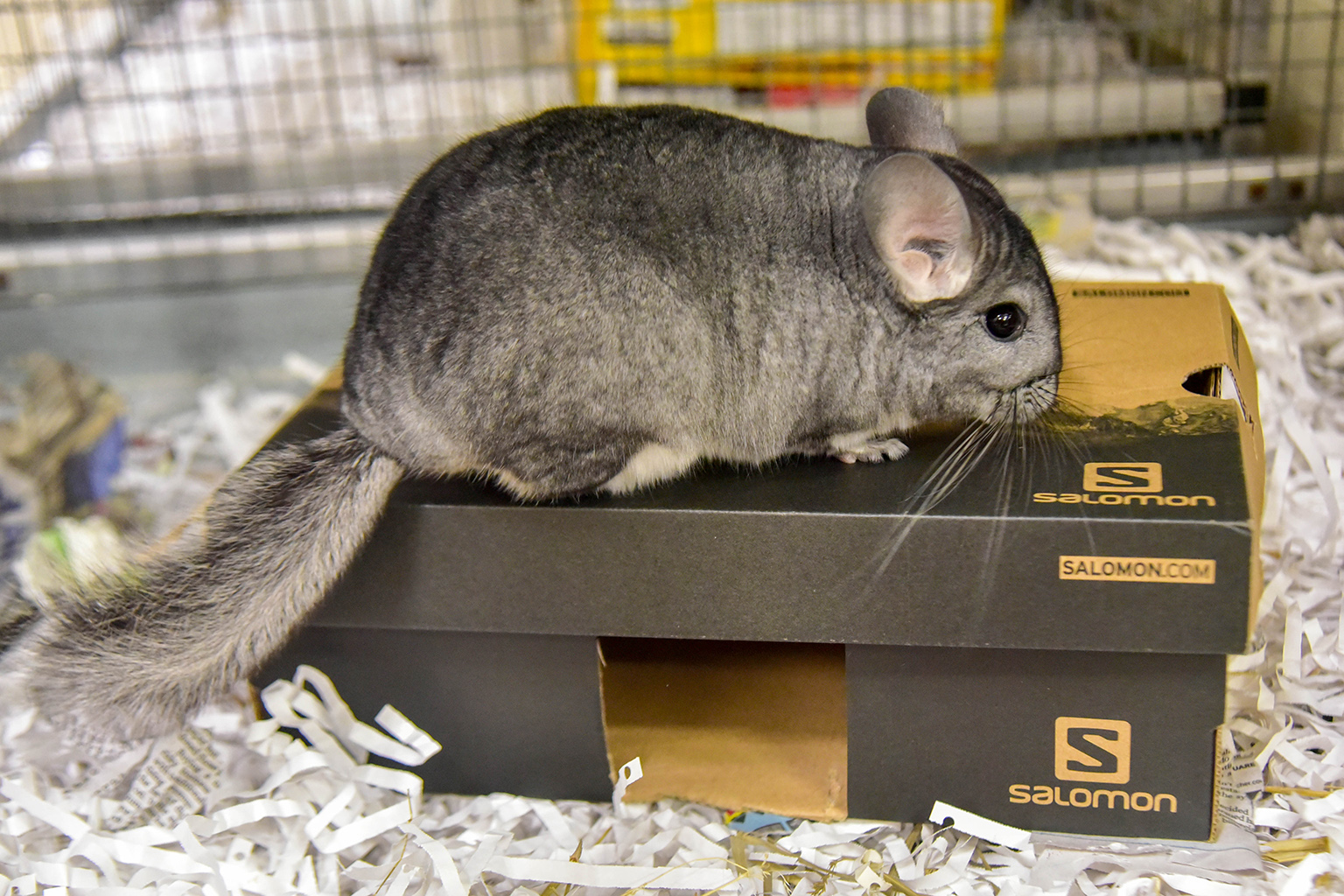In the image, a pet dormouse is enclosed in a cage, sitting atop a Salomon shoebox, which serves as its makeshift house. The shoebox is gray with yellow accents and has a hole cut into the side, likely for the dormouse to enter and exit. The dormouse has a robust, gray body interspersed with black hairs, large black eyes, long whiskers, and notably big ears. It also sports a bushy tail, quite different from the usual long, rubbery tail of a common mouse, and its face appears flatter and rounder. Shredded white paper covers the floor of the cage, providing bedding and burrowing material for the dormouse. The dormouse, which is surprisingly large, comparable to a woman's size seven or eight foot (approximately eight to nine inches), looks a bit apprehensive with its wide eyes. In the background beyond the cage, there are indistinct boxes or perhaps other cages.